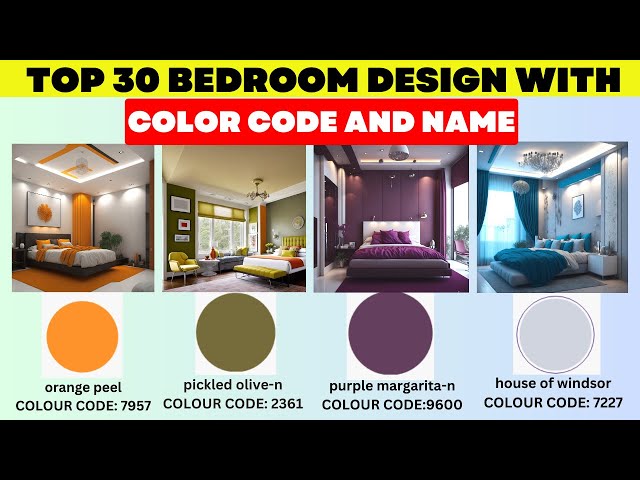The image displays an informational advertisement set against a black background with solid black borders on the top and bottom. At the top, a bold yellow banner with black text reads "TOP 30 BEDROOM DESIGN WITH," followed by a red banner with white text reading "COLOR CODE AND NAME." Below these banners, four different bedrooms are showcased, each styled distinctively with varied color schemes and decor elements. The bedrooms have tall ceilings and formal appearances. The first bedroom, highlighted with orange decorations, is labeled "Orange Peel," accompanied by a small orange circle and color code 7957. The second bedroom features green decor and is labeled "Pickled Olive," with a small green circle and color code 2361. Following that, the third bedroom showcases purple accents, labeled "Purple Margarita," with a purple circle and color code 9600. The fourth bedroom displays blue themes, titled "House of Windsor," marked by a light blue circle and color code 7227. This detailed layout presents a visually appealing guide to varied bedroom designs and their specific color identifications.